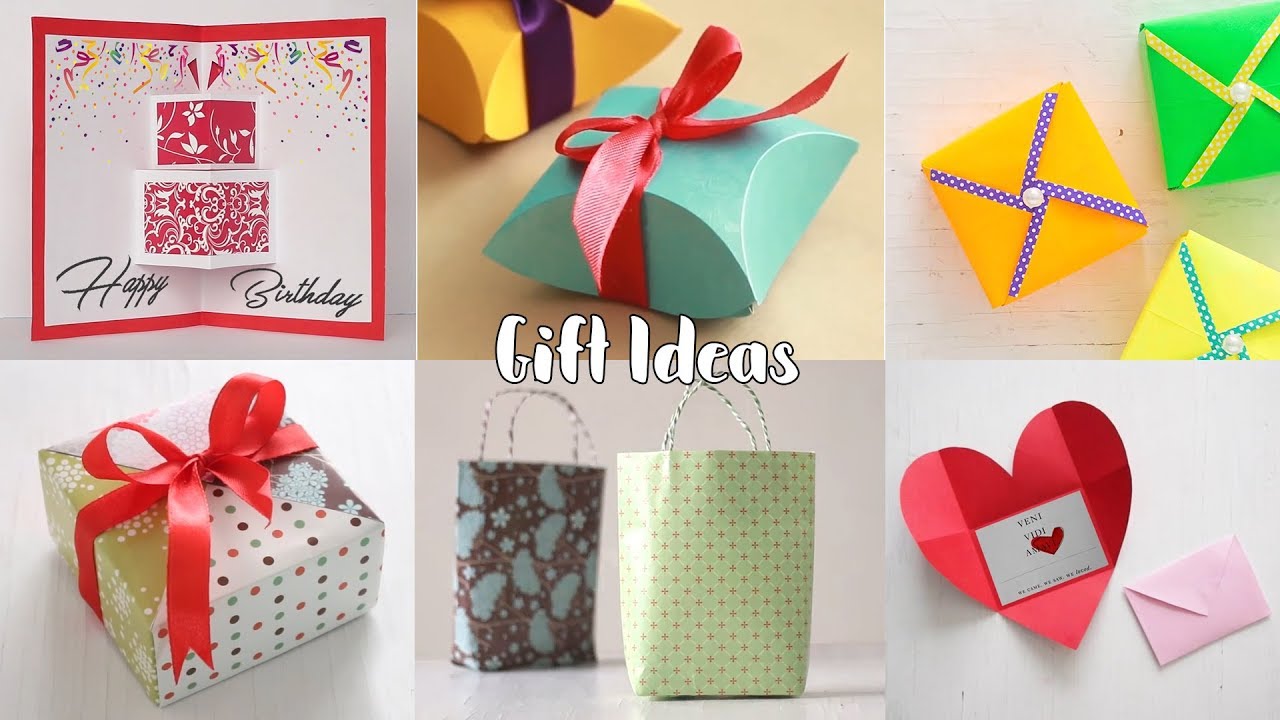The image is a rectangular, colored collage divided into six sections with two rows of three images each, centered around a white, block-style font that reads "Gift Ideas" outlined in black. The top row begins with an open "Happy Birthday" card decorated with a pop-up cake and a red border. Next is a small, square, turquoise box tied with a neat red ribbon bow. The third image in this row features three colorful gift boxes—orange, green, and yellow—arranged in a simple design on fabric lines, pinned at the middle with a push pin. Moving to the bottom row, the left-side image showcases a traditionally wrapped gift box with multicolored wrapping paper and a red bow. The middle image displays two patterned gift bags, one blue and brown, the other green with stars. The final image in the bottom row shows a heart cut out of paper, resembling a school crafting project, accompanied by a pink envelope. The heart has visible folds and inscribed with the text "Veni Vidi We Came We Saw We Loved."